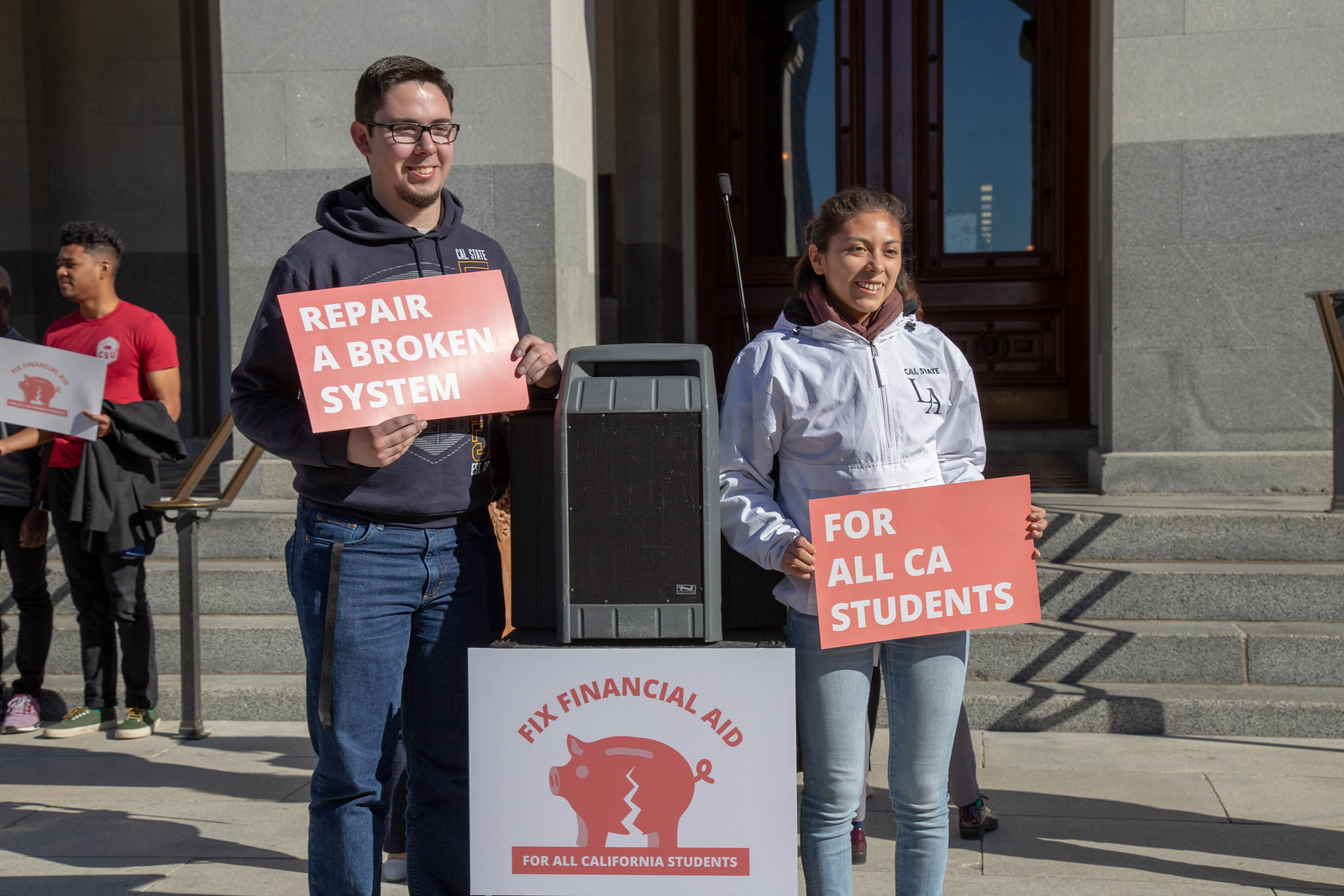In front of a large gray municipal building with old brown doors and windows, several people are gathered, seemingly participating in a political rally or protest. Prominently in the foreground, a man on the left is holding a red sign that reads "Repair Your Broken System." He is wearing a gray sweatshirt, jeans, and rectangular black glasses, with a name tag partially visible from his right pocket. Beside him, a woman in a light gray sweatshirt with a brown collar holds a matching red sign that says, "For All CA Students." She has her hair pulled back and wears light blue jeans. Between them stands a gray and black speaker with a sign propped on it, displaying "Fixed Financial Aid" above an image of a damaged piggy bank, underneath which reads, "For All CA Students." In the background to the left, a man can be seen wearing a red shirt and dark pants, while another person stands nearby, contributing to the sense of collective action on this clear, sunny day.